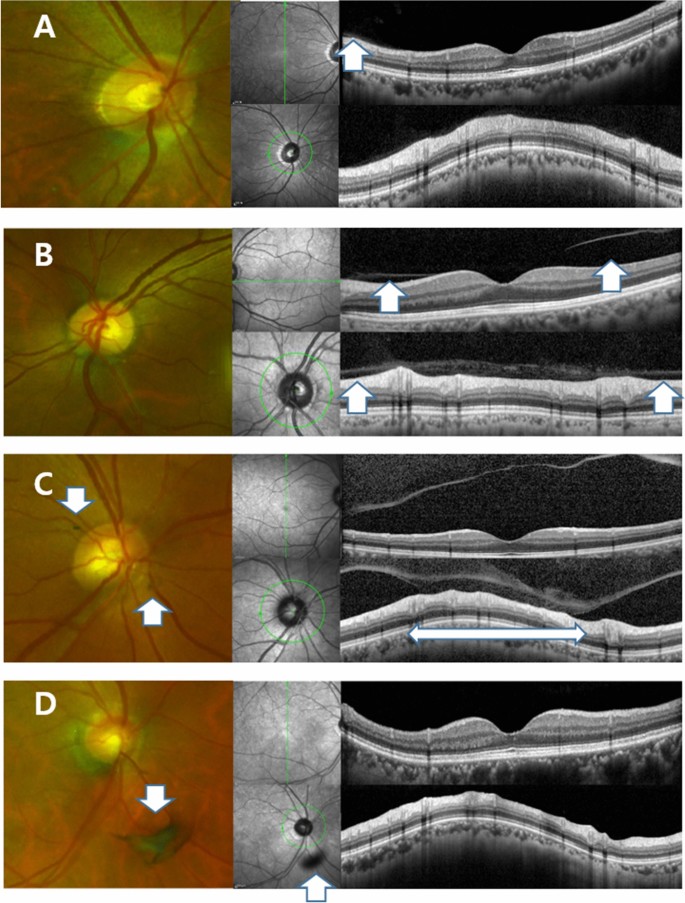The image comprises a series of four horizontal sets of medical images labeled A, B, C, and D, arranged from top to bottom. Each set consists of three distinct images. The first image in each set is a colored picture showing an anatomical structure with a yellow background and red veins, encased in a green outline, which resembles an eyeball or a similar organic structure. To the right of the colored image, there are two black and white images; the first is a vertical rectangle presenting the same structure in grayscale, and the second is a horizontal rectangle showing a related feature, likely an artery or blood vessel, from a different angle. Each set also includes arrows of various colors pointing to specific regions within the images to highlight important areas. This detailed arrangement seems to be diagnostic in nature, possibly utilizing techniques like x-rays or CAT scans to capture varying views and perspectives of the anatomical features.